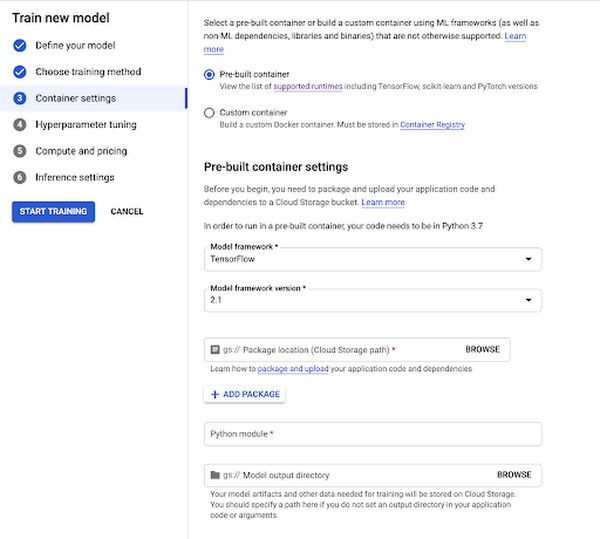**Detailed Caption:**

The image displays a comprehensive guide for setting up and training a machine learning model, segmented into two columns against a predominantly white background.

**Left Column:**
1. **Header:** "Training Model"
2. **Task List:**
   - **Completed Tasks** (indicated by check marks):
     - Define your model
     - Choose training method
   - **Pending Tasks**:
     1. Container settings
     2. Hyperparameter tuning
     3. Compute and pricing
     4. Insurance settings
3. **Footer**: Contains a button labeled "Stop Training" with an option to cancel the training process.

**Right Column:**
1. **Information Section:**
   - **Guidance on Containers**:  
     "Select a pre-built container or build a custom container using MI."
     - Options provided:
       - Pre-built container
       - Custom container
     - Descriptions of each option.
   - **Pre-built Container Settings** (in bold):
     - "Before you begin, package and upload your application code and dependencies to a cloud storage bucket."  
       (Includes a "Learn more" link)
2. **Requirements:**
   - "To run a pre-built container, your code must be in Python 3.7."
3. **Options to Select:**
   - "Framework" drop-down menu with selectable options
   - "Framework version" drop-down menu with selectable versions
4. **File Management:**
   - **Package Location:**
     - Field to input the cloud storage location, including a "Browse" option.
   - **Add Packets Section:**
     - Button with a plus sign for adding packets.
5. **Model Directory:**
   - **Python Model Box**: Field to input the Python model.
   - **Model Output Directory**: Includes a browse option and a descriptive paragraph explaining its usage.

The overall setup provides an in-depth walkthrough for configuring various settings and uploading necessary files for training a machine learning model using the outlined methods.